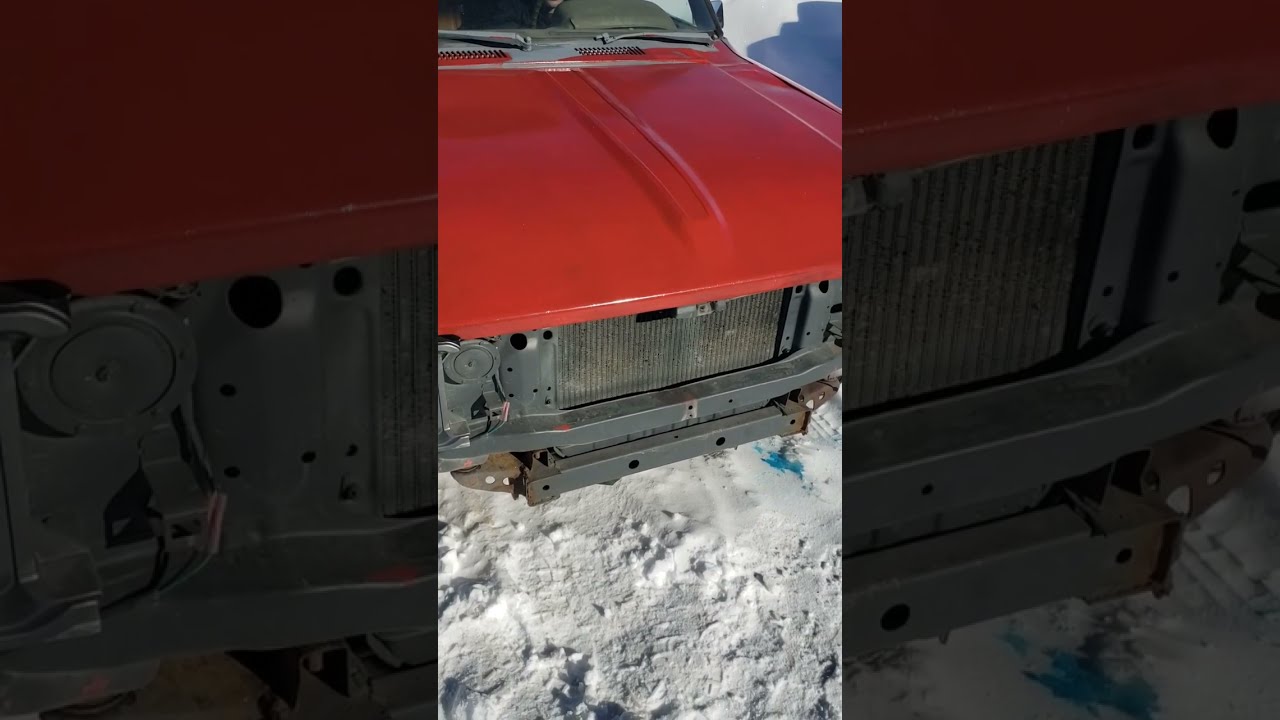The image is a digital photograph, likely a vertical format akin to a TikTok video, depicting the front side of an older car, possibly a muscle car from the 1970s. The car is predominantly red, especially the hood which features a raised indentation down its middle. The car rests in a snowy environment, with the ground blanketed in snow but the car itself free of it. Notably, the vehicle is missing its front grille and bumper, exposing the radiator and other internal mechanical components. The front fender is also absent, revealing more of the car’s inner structure, including some wires and black sections of the body. Windshield wipers are visible, though the headlights and grille are missing. The snow around the car is slightly dirty and has embedded bits and grasses, suggesting it’s been there for a while. Snow in the vicinity shows no signs of footprints, contrary to another part of the description which implies that there might be small prints in the snow. Additionally, there is a noticeable blue fluid leaking from the car on the right side of the image, further indicating its neglected state. The overall color palette includes red, black, rust, white, and gray, with some charcoal gray in the exposed grille area and the leaking blue fluid providing a stark contrast.